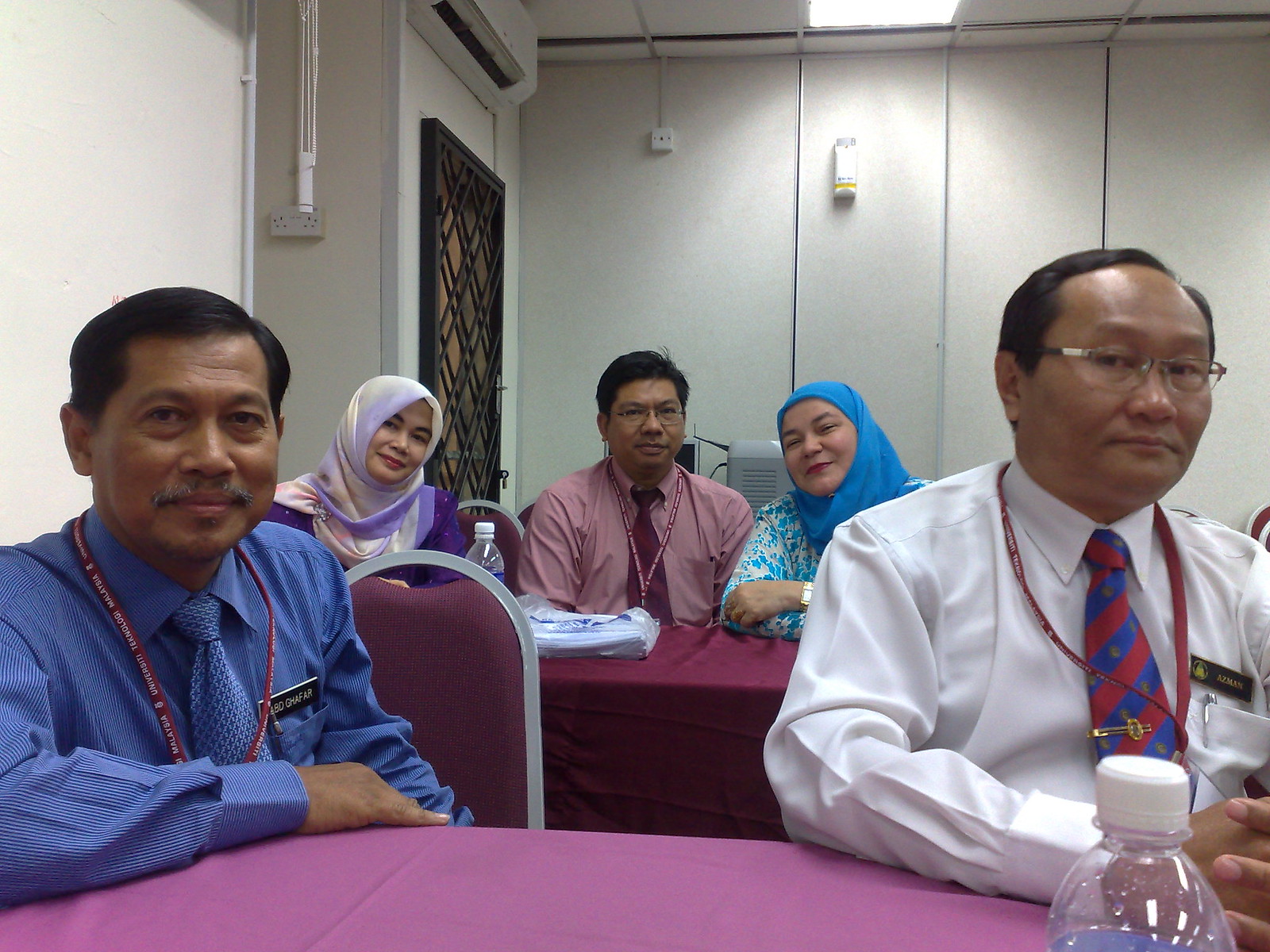Five participants are seated at tables in what appears to be a small conference or meeting setting. The men, adorned with neck bands bearing ID tags—though unreadable—suggest some type of conference or special access. Seated in an arrangement that indicates they are either waiting to listen to or already listening to a speaker, the participants display a mix of attentive and contemplative expressions.

Starting from the left, a man in a blue sports shirt and matching blue tie wears an unreadable name tag. On the far right, another man is dressed in a white shirt paired with a blue and red tie, accentuated by a gold tie clasp and a pen clipped to his pocket—identity also obscured by an unreadable name tag. 

At the back, front and center, sits a man in an off-red or off-tan sports shirt, paired with a light contrasting tie. He is flanked by two women, each wearing headscarves. The woman to his right dons a blue headscarf, while the woman to his left sports a multicolored pastel headscarf. 

An assortment of personal items, including a water bottle, are spotted on the tables adorned with reddish tablecloths, in a bright room with a tile ceiling. The environment features a modular air conditioner and visible wall switches and a thermostat, enhancing the room's functional aesthetic. The participants' attire and features suggest a Southeast Asian origin, possibly Malaysia, enhancing the cultural bedding of this intimate and focused gathering.